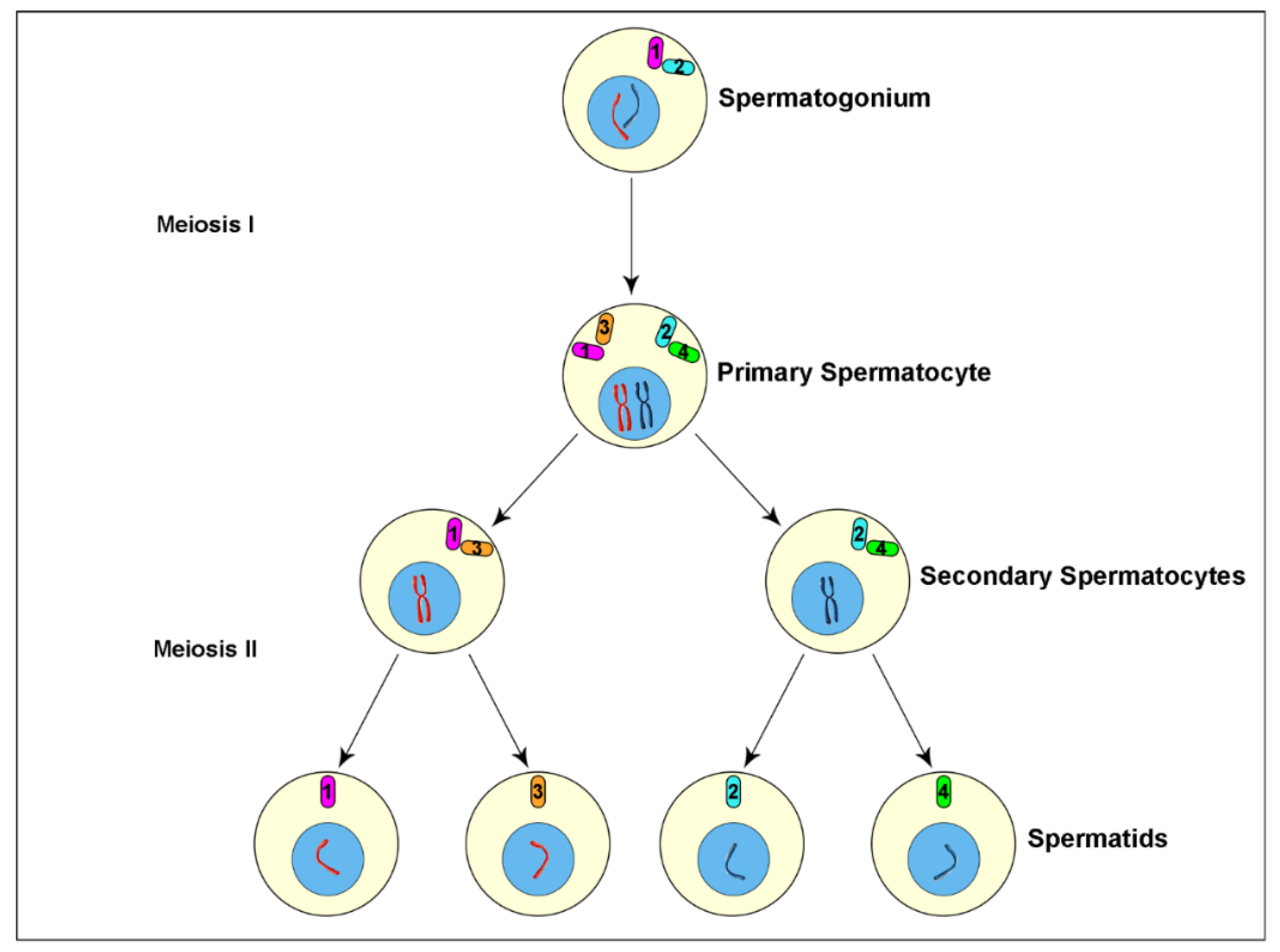This infographic poster, set against a white background with a thin black border, presents a detailed flowchart of genetic inheritance and meiosis. The illustration is in color with black text, displayed in landscape orientation. On the left side, two labels demarcate stages: "Meiosis 1" at the top and "Meiosis 2" at the bottom. 

At the apex of the chart is a circle labeled "Spermatogonium," which holds two blue squiggles inside. An arrow points downward to another circle labeled "Primary Spermatocyte," also containing a blue circle with two squiggles. This circle branches diagonally into two circles labeled "Secondary Spermatocytes," each with an X chromosome shown in blue.

From these secondary spermatocytes, arrows branch further into four circles at the bottom of the chart. These circles, labeled "Spermatids," are numbered 1 through 4 and each contains a smaller blue circle with a unique squiggle pattern, indicating different chromosomal configurations in red or blue.

The entire poster uses a pyramid-like structure to illustrate the sequential stages of meiosis and sperm development, starting from the single spermatogonium at the top and culminating in the four spermatids at the bottom. This color illustration efficiently conveys the complex process of genetic inheritance through the use of detailed annotations and clear, structured arrows.